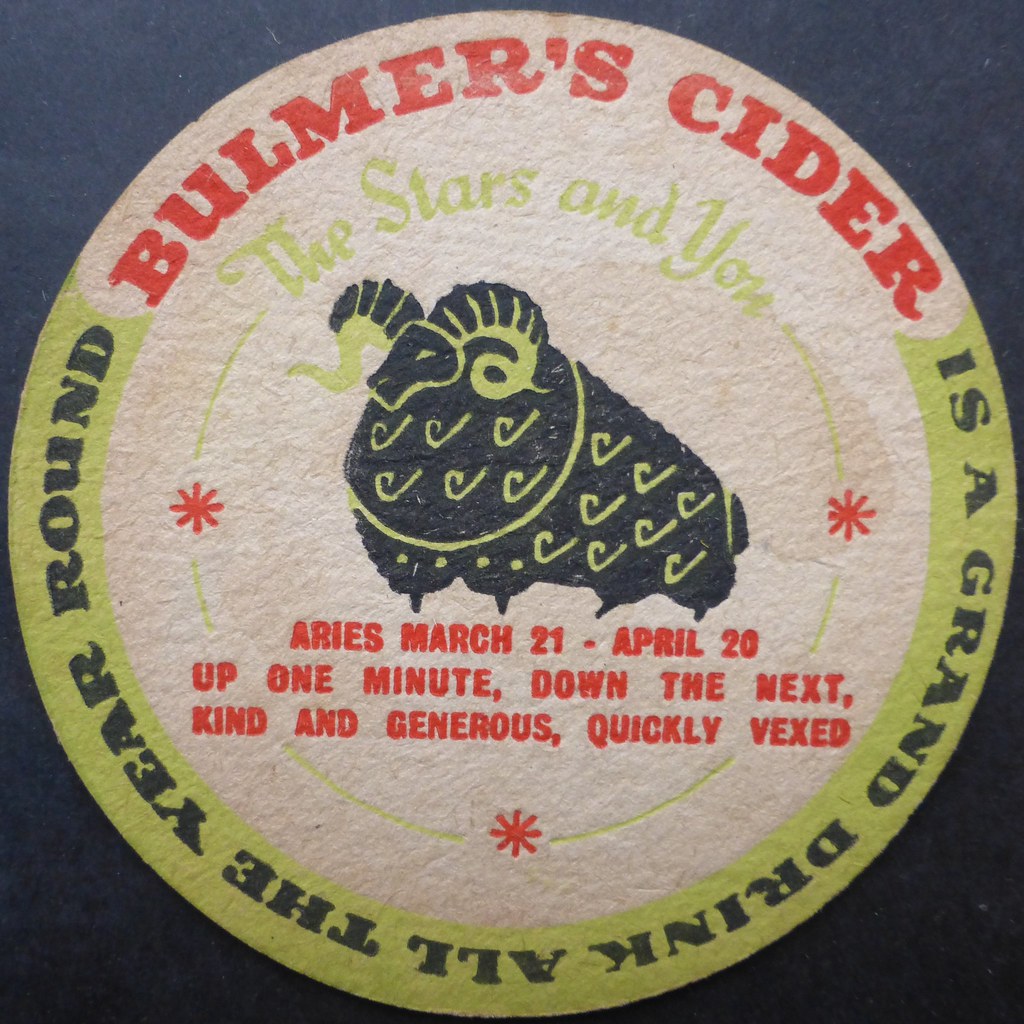The image displays a round ad for Bowmer's Cider, possibly a drink coaster, set on a dark blue table or countertop. At the top of the circle, in red text, it reads "Bowmer's Cider." Encircling the bottom half in black letters on a green background, it states, "is a grand drink all the year round." Inside the circle, just beneath "Bowmer's Cider," it says, “The Stars and You” in green. Central to the design is an illustration of a ram with rounded horns, labeled "Aries, March 21st to April 20th" below in red text on a white background, along with the words "up one minute, down the next, kind and generous, quickly vexed." The ram is flanked by three asterisks, enhancing the visual symmetry of the ad.